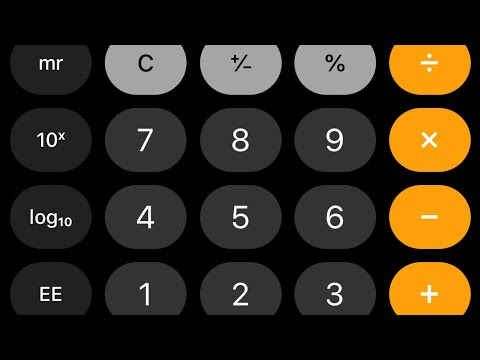This image is a detailed computer animation screenshot of an up-close section of a scientific calculator, set against a black background. The interface is divided into four distinct rows, each containing five oval-shaped buttons. 

In the first row, starting from the left:
- The first oval is black, labeled "MR".
- The next three ovals are light gray. The first light gray oval features a "C", the second one displays a "+/-" sign, and the third is marked with a "%".
- The last oval in this row is yellow with a division symbol (÷).

In the second row:
- The first button is black and marked with "10^x".
- The subsequent three buttons are a slightly lighter gray and labeled "7", "8", and "9" respectively.
- The final oval in this row is yellow with a multiplication symbol (×).

In the third row:
- The initial button is black featuring the label "log" with a "10" subscript at the bottom right of the 'g'.
- The next three buttons, which are also in lighter gray, are numbered "4", "5", and "6".
- The last button in this row is yellow with a subtraction symbol (−).

In the fourth and bottom row:
- The first button is black and labeled with "EE".
- The next three buttons are a dark gray, numbered "1", "2", and "3".
- The final button in this row is yellow, adorned with an addition symbol (+).

The detailed labeling and varied coloration of the buttons highlight the multifunctional aspects of this scientific calculator.